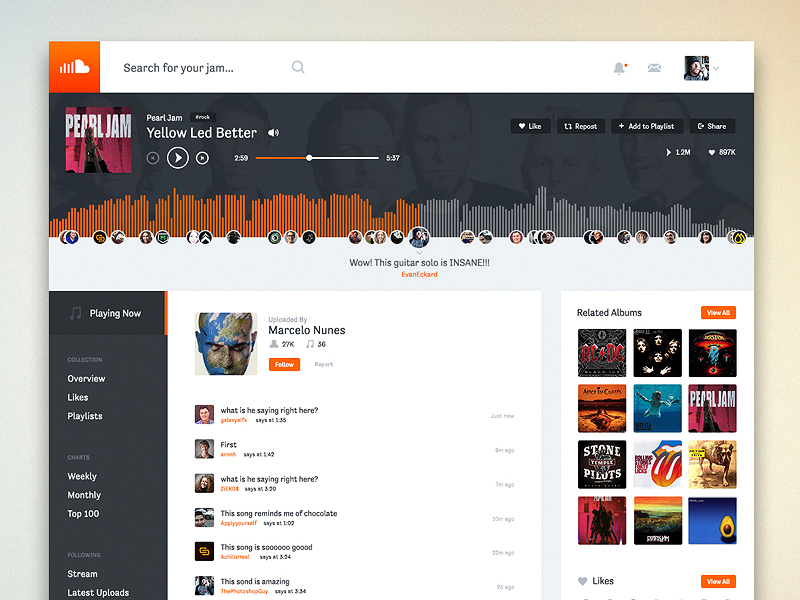**Caption:**

The profile view showcases a vibrant mix of music and user activity. Dominated by SoundCloud aesthetics, the profile features an array of orange squares and clouds, contributing to its lively interface. Highlighted tracks include "Stitchfield Jam" and "Ramp Sunglass," along with iconic bands like Pearl Jam, whose song "Let It Bitter" stands out in yellow. 

User reactions are enthusiastic, with likes and reposts emphasizing the popularity of the songs. Comments spotlight an insane guitar solo by Evan Eckhart, prompting exclamations such as "Wow!" Currently playing is a collection overview that includes likes, playlists spanning weekly and monthly top 100, and streams. Additional sections feature the latest uploads and Marcella News follow-up reports.

A noticeable comment reads, "this song reminds me of chocolate, this song is so good," further highlighting the user engagement. Related albums and artists are recommended, featuring legends like ACDC and Queen, alongside vibrant visuals of a dog, varying color squares, and blue elements, creating an engaging and dynamic musical experience.